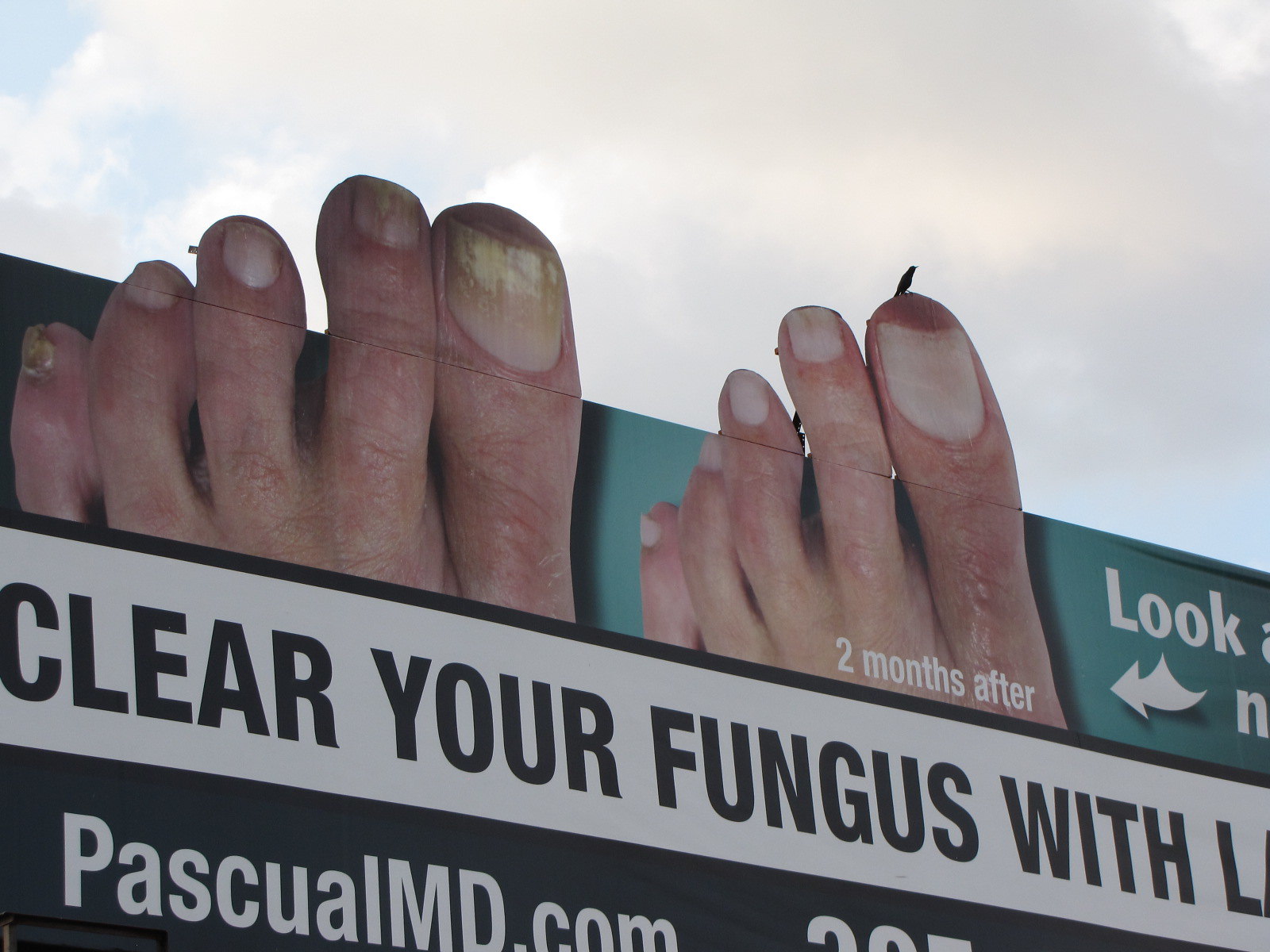The image is a photograph of an old-style billboard advertisement viewed against a backdrop of a blue sky with puffy white clouds. The advertisement prominently features before-and-after pictures of two right feet, showing the effects of a foot fungus treatment. The "before" image on the left displays nails with distinct discoloration and unhealthy appearance, while the "after" image on the right shows noticeably healthier, fungus-free nails, labeled as "Two Months After." The billboard prominently reads "Clear Your Fungus" in black letters, with an arrow pointing towards the treated toes. Below this, a white banner displays the text "pasqalmd.com" in white letters, though part of the contact information is cut off. Adding a whimsical touch, a bird is perched on one of the toes. This advertisement, set against a bright, cloud-filled sky, aims to promote a podiatrist's services for treating foot fungus.